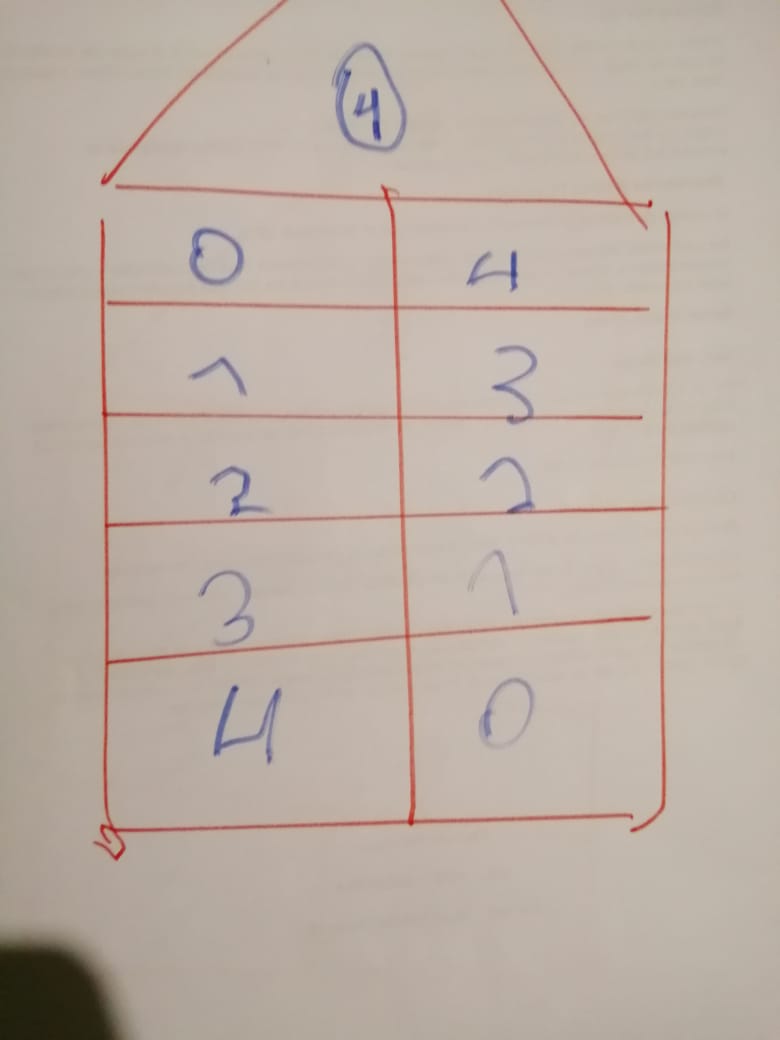This photograph features a meticulously drawn grid pattern using red marker, against an off-white, almost light gray background. The grid resembles the layout of a building with five distinct stories, topped by a triangular section that evokes the image of a roof. This triangle at the top houses a circled number "4" written in blue marker, indicating a focal point. The grid itself is sectioned into what appear to be rooms, each marked with blue numerals that vary in clarity, suggesting the blue marker is running out of ink.

The floors are detailed as follows: the top triangular section contains a circled four, the fifth floor features the numbers zero and four, the fourth floor has a slanted seven and a three, the third floor is marked with two and a two, the second floor displays a three and a seven, and the first floor shows four and zero. The entire grid and triangle are clearly outlined in red marker, contrasting with the fading blue numbers which indicate specific scores or planning notations for a game.

A subtle shadow is present in the bottom left corner of the image, possibly cast by an individual standing nearby, partially obscuring the light. This shadow adds a hint of depth to the otherwise flat, schematic drawing.